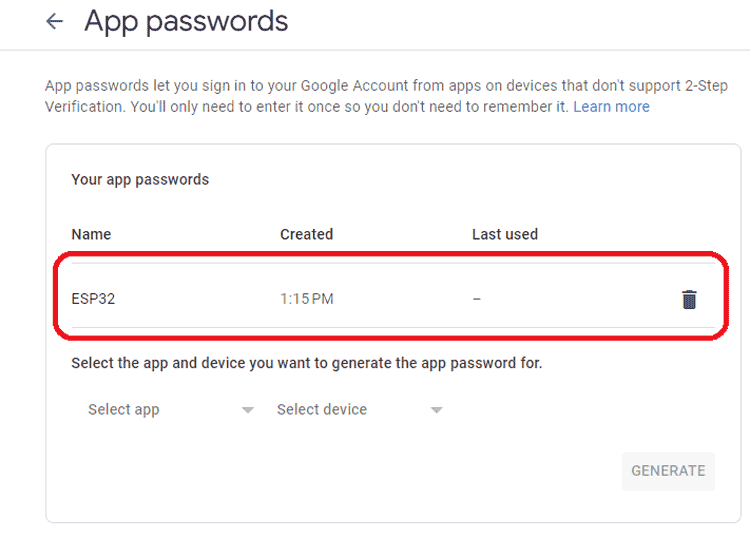A screenshot displays a detailed view of the Google Account settings, specifically the "App Passwords" page. This setting is used for applications and devices that do not support Google's two-step verification. The header of the page explains that app passwords enable users to sign into their Google Account from such apps and devices without needing two-step verification each time. Instead, users enter the app password once, and it eliminates the need to remember it thereafter. There is a "Learn more" link provided for additional information.

Beneath this explanation, an entry is shown for an app named "ESP32," which was created at 1:15 PM but has never been used. This is indicated by a dash under the "Last used" column. To the right of this entry, there is a trash can icon, suggesting that users can delete the app password if desired.

For those who wish to add more app passwords, there are instructions to scroll down, select the appropriate app and device from the dropdown menus, and then click the "Generate" button located at the bottom right of the page. The caption summarizes that this Google setting allows users to bypass the typical two-step verification process for certain apps and devices, facilitating easier access while maintaining a level of security.